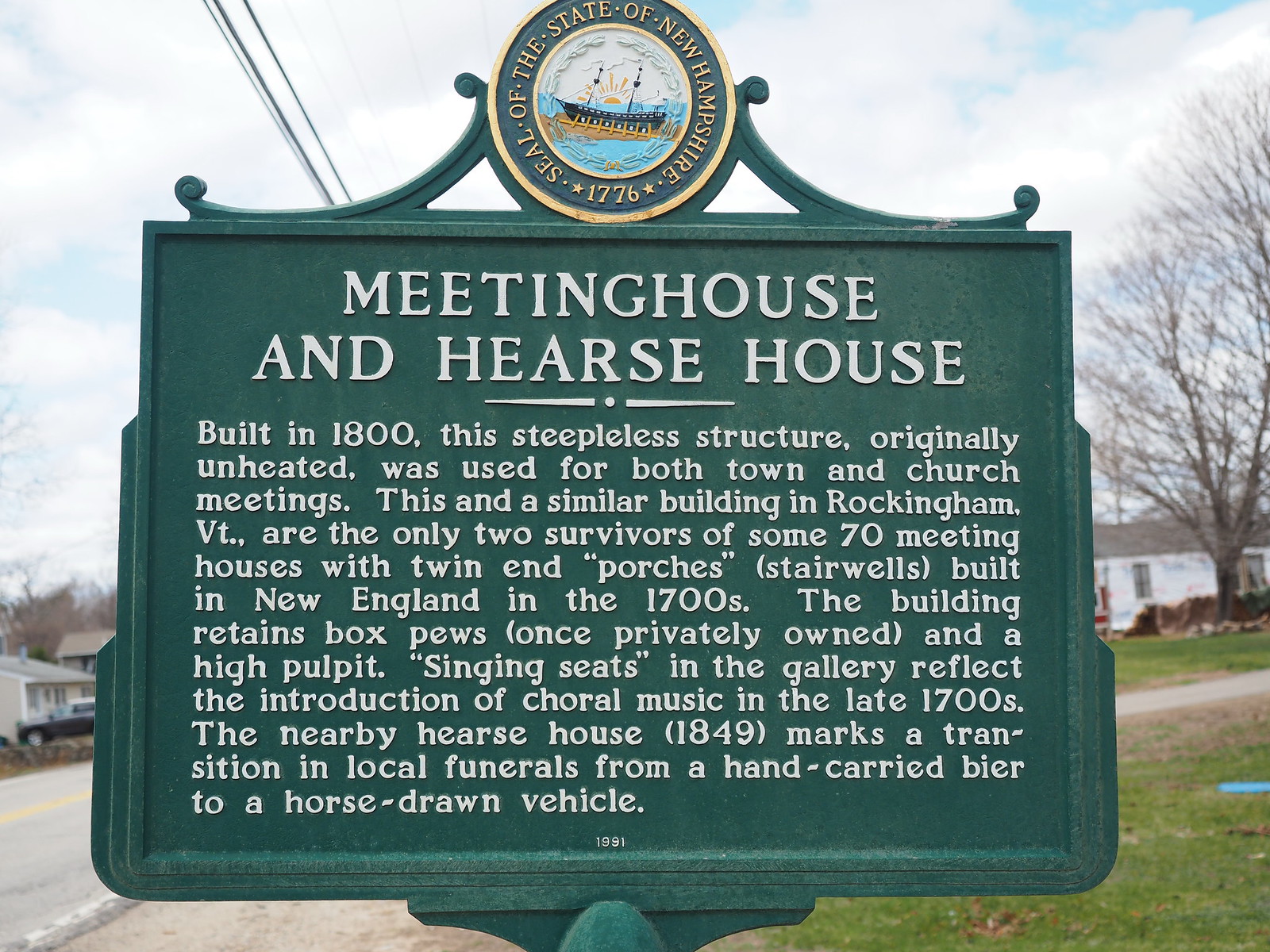This image, taken outside during the daytime, shows a historical sign standing on a green grassy area. The dark green metal sign, slightly wider than it is tall, features a gold-outlined circular seal at the top reading "Seal of the State of New Hampshire 1776," depicting a ship with the sun behind it. Below the seal, in large white letters, the sign is titled "Meeting House and Hearst House." It details that the Meeting House, built in 1800, is a steeple-less structure originally unheated and used for both town and church meetings. It notes that this building, along with a similar one in Rockingham, Vermont, are the only two surviving of the approximately 70 meeting houses with twin-end porches and stairwells built in New England during the 1700s. The Meeting House retains box pews, once privately owned, and a high pulpit, with singing seats in the gallery reflecting the introduction of choral music in the late 1700s. The nearby Hearst House, built in 1849, marks the local transition of funerals from hand-carried biers to horse-drawn vehicles. The scene behind the sign includes a partly cloudy sky with patches of blue, telephone poles, electric lines, a street to the lower left corner with a house behind it, and a yard with a tall tree on the lower right side.